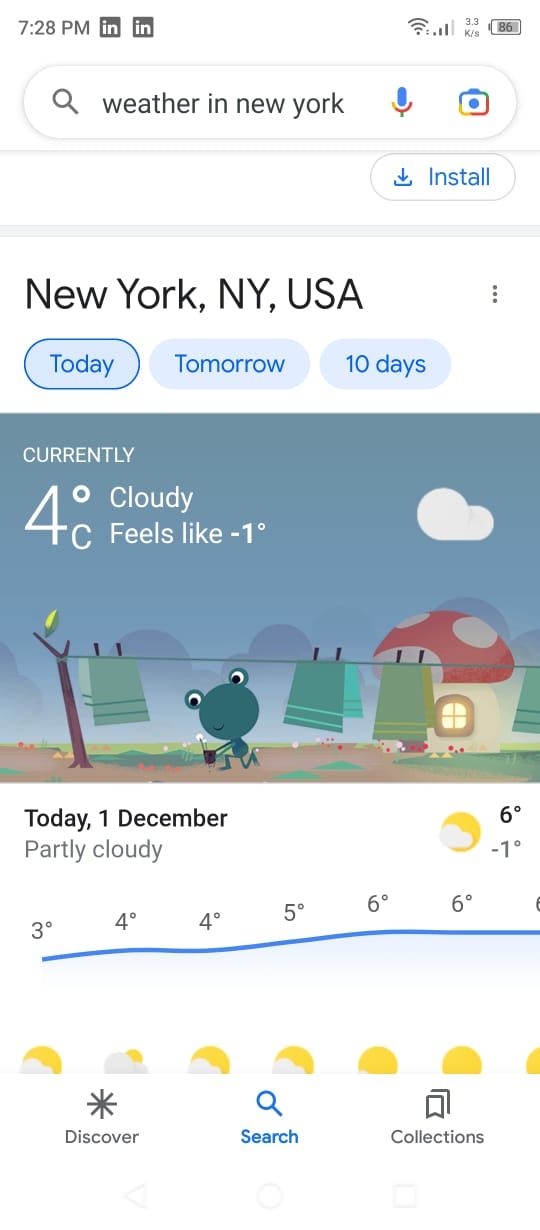The image is a phone screenshot of a Google search for the weather in New York. At the top right, the phone's battery icon shows 86% charge. Next to it, there is download information displaying 3.3 K/S, and to the left of that, the phone signal strength is at three bars along with full bars for Wi-Fi. The top left corner indicates the time of the screenshot was 7:28 PM, accompanied by two LinkedIn icons.

Below the status icons, the search bar is visible with the query "weather in New York." To the right of the search bar, there are colorful blue, yellow, and red icons for the microphone and the camera. Below the search bar, there is an install button and another button likely for downloading or sharing.

In the middle of the image, it prominently displays "New York, New York, USA," followed by three tab options: "Today," "Tomorrow," and "10 days." Under these tabs, it shows the current weather as "4°C, cloudy, feels like -1°C." A whimsical graphic depicts a frog planting in a pot, sitting in front of three clouds.